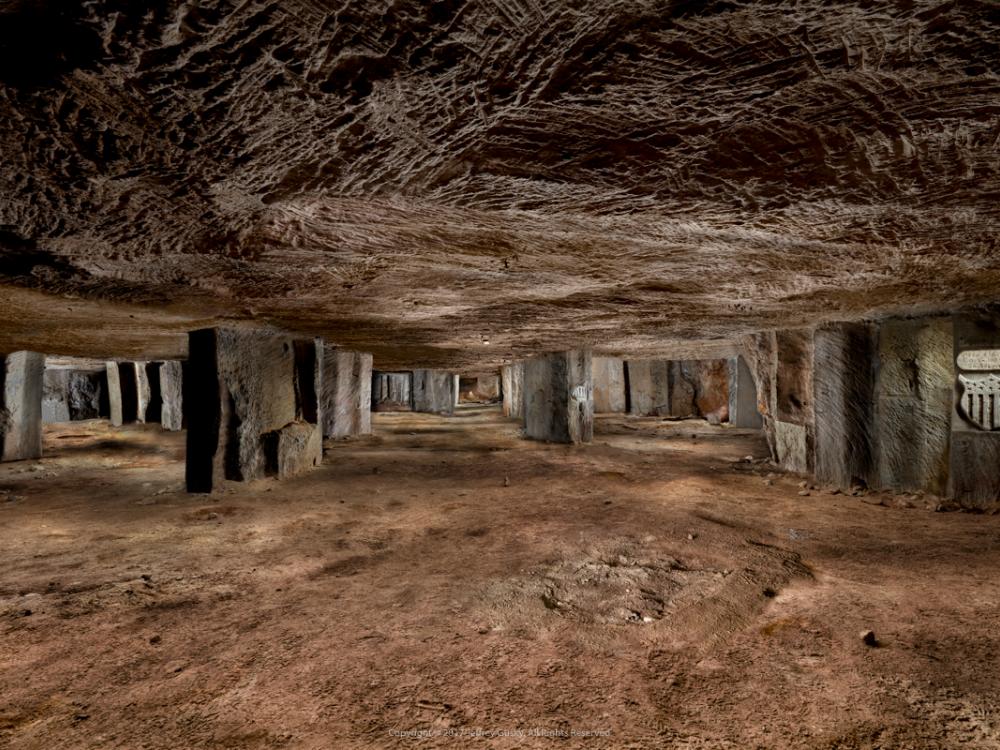This digital landscape photograph depicts an underground scene that resembles a cave or a substructure. The ground, extending from the bottom left to the bottom right, is a mix of light brown dirt and sand, riddled with patches and holes. The ceiling above, which spans from top right to top left, appears to be a thatched or rocky surface, supported by large, rectangular stone columns. These columns create an impression of multiple pathways extending into the distance. The earthy tones of brown and grey dominate the scene, contributing to its rugged and ancient appearance. A small, barely legible white print at the very bottom contains what seems to be a copyright notice, ending with "all rights reserved." Near the right side of the image, there's a peculiar metal indentation resembling a shield, accompanied by a plaque. The overall ambiance is one of an expansive, abandoned underground passage, filled with natural textures and structures.